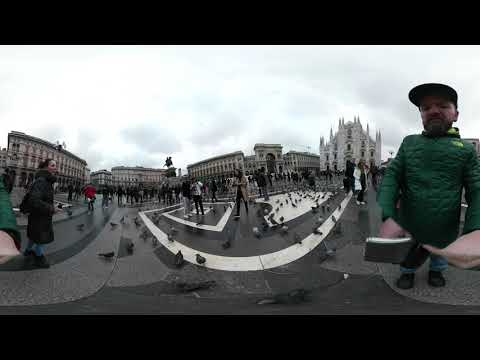The image captures a bustling outdoor scene, likely at a tourist destination in a European city. Taken with what appears to be a 360-degree or concave lens, the photograph has a slightly warped and low-resolution quality, but it remains rich in detail. In the foreground, the stone ground, composed of gray and black tiles with white patterns, is teeming with dozens of black pigeons. The right side of the image features a bearded man dressed in a green jacket and a dark hat, possibly the photographer, who might also be a tourist guide; he's facing the camera and holding an object in one hand while extending the other. On the left, a woman in a long black coat looks towards the right side of the image, adding to the dynamic scene. The background reveals a large crowd scattered across the area, engaged in walking and picture-taking, suggesting a cold day due to their heavy jackets. An ornate, white-colored building with multiple spires, possibly a church, can be seen in the middle distance just left of the man, extending upwards and flanked by several other older, ornate buildings constructed from brown stone or brick. The sky overhead is dark and heavily clouded, casting a muted light over the entire scene.